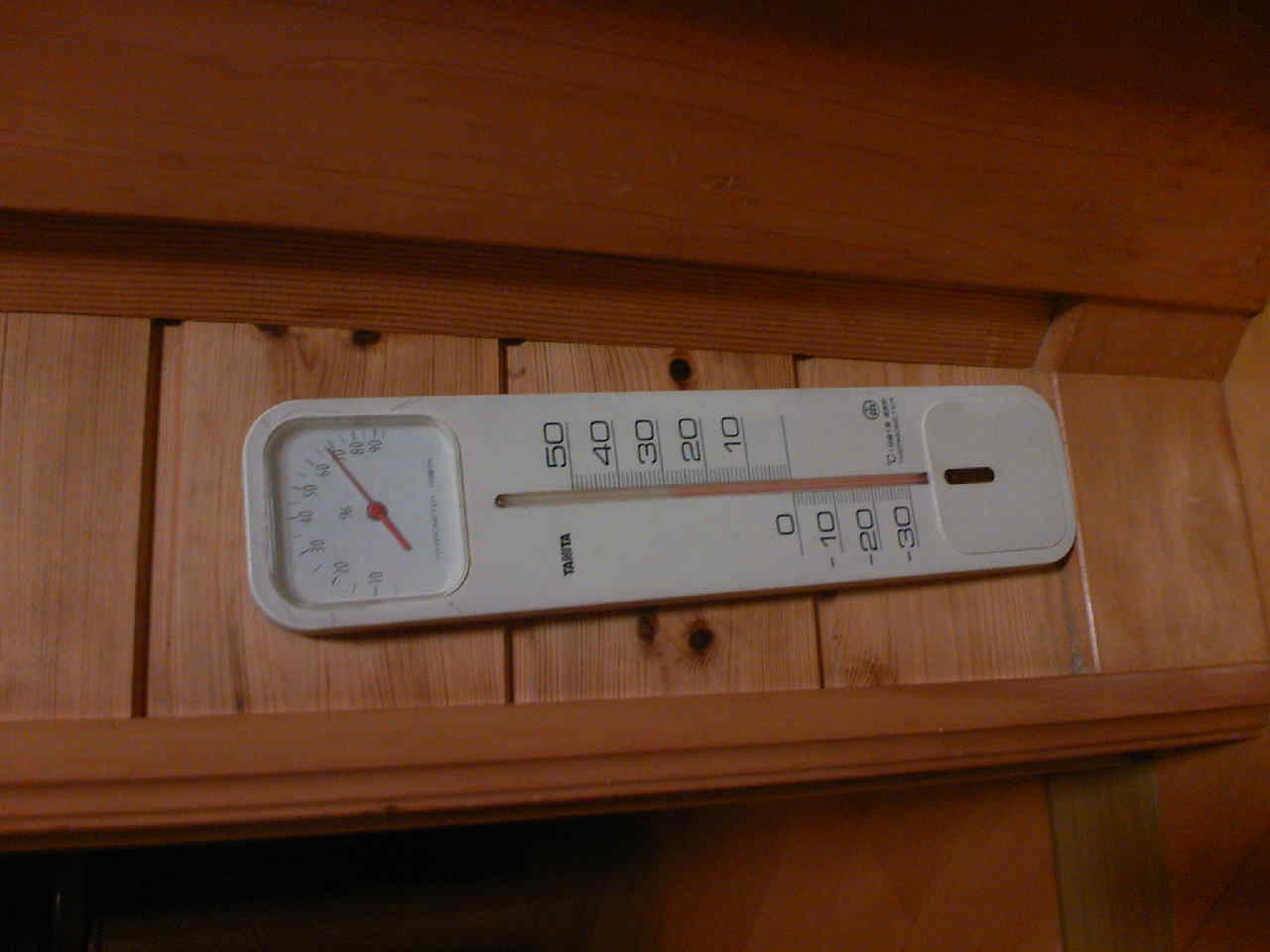In this horizontally-oriented photograph, an old-fashioned mercury thermometer is prominently displayed against a backdrop of wooden planks. The thermometer, mounted horizontally, has its gauge starting from 10 degrees on the left, escalating by tens up to 90 degrees on what is typically the top side. Additionally, it shows a reverse scale of 50, 40, 30, 20, 10, reaching down to 0 and further into negative values of minus 10 to minus 30 degrees. The thermometer features a red indicator hand and red mercury within a white frame, secured to cedar-colored shiplap panels. This setup appears to be at the entrance of a rustic sauna, with the sauna room visible at the bottom edge of the photograph due to its sideways orientation. Unreadable text accompanies the numbers on the right side of the thermometer, adding an element of aged authenticity to the scene.